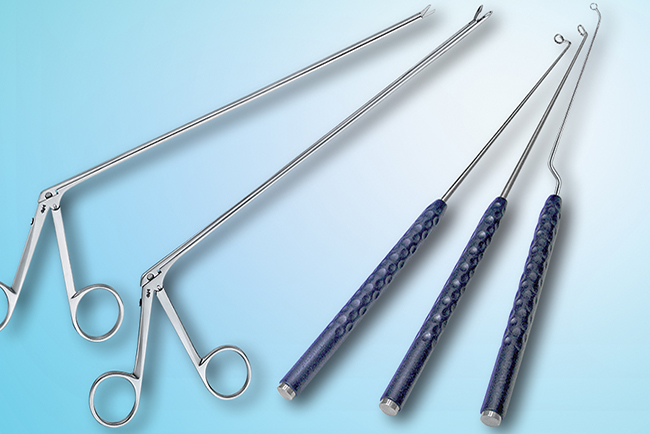The image depicts a collection of five medical instruments arranged side by side against a gradient background of light cyan blue fading to white at the top right. On the left side of the image, there are two identical scissor-like instruments, featuring long, extended metal arms that lead to clipping mechanisms designed for cutting or trimming tissue. These instruments appear to be stainless steel and are likely used for precise surgical applications. On the right side, there are three similar-looking tools with long probes ending in tiny metal loops. These tools have blue, dimpled handles for a secure grip, which suggest they might be used for scraping plaque off teeth or for other delicate procedures requiring precision, possibly even in deep body cavities. Each tool is meticulously arranged to showcase its design and function, highlighting the specialized nature of these surgical instruments.